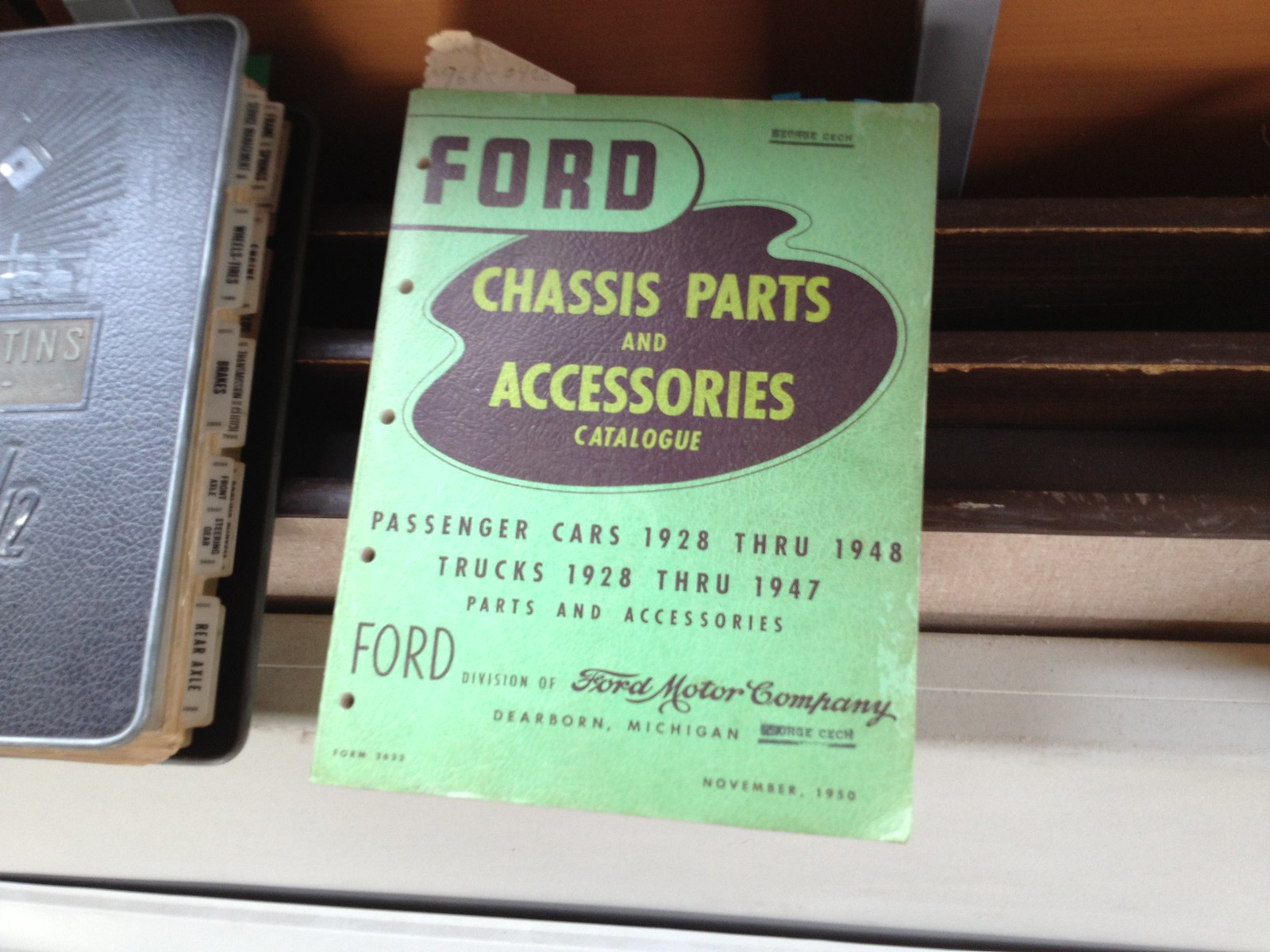The image shows a well-worn Ford Chassis Parts and Accessories Catalog, released in November 1950, prominently featuring a teal or lime green cover. The catalog is titled in black and yellow lettering, indicating it covers Passenger Cars from 1928 through 1948 and Trucks from 1928 through 1947, and is issued by the Ford Motor Company in Dearborn, Michigan. The catalog is visually distinct with its detailed design and historical value, making it a standout piece. To the left of the catalog is a leather-bound book with an embossed cover, which is properly indexed but with unreadable titles due to the way it's positioned. The setting appears to be a rustic wooden shelf, suggesting a used bookstore or perhaps a vintage library, with a noticeable white bookmark sticking out of the catalog. The background includes a hard surface with some sort of railing or bars, adding an additional layer of texture and depth to the scene.